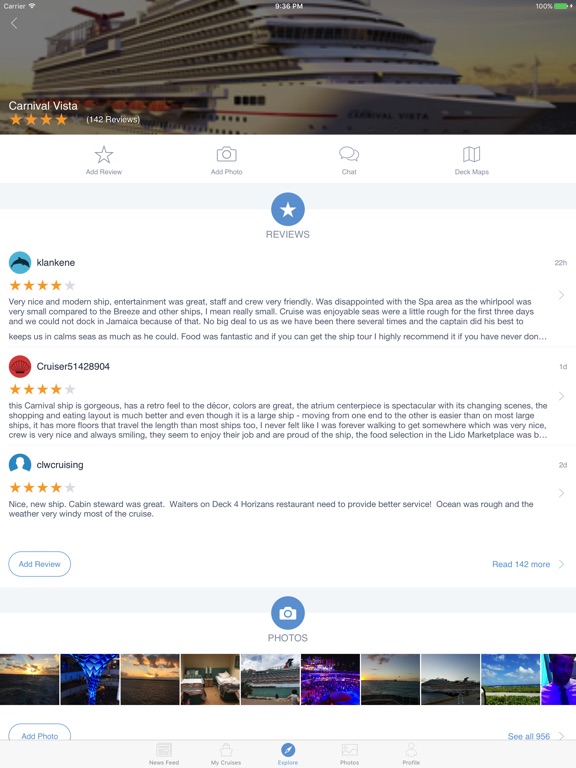This is a screenshot of a website page dedicated to the Carnival Vista cruise ship. The top portion of the image, occupying less than a quarter of the screen, prominently features a large photograph of the Carnival Vista, showcasing its expansive multi-story design. Just below the photo, on the left, the text "Carnival Vista" is clearly visible, accompanied by four orange stars and a note indicating 142 reviews.

Below this, a navigation strip includes options labeled "Add Review," "Add Photos," "Chat," and "Doc Maps." Central to this section is a blue circle with a white star icon, next to which the word "Reviews" is displayed. Three individual reviews are listed beneath this heading. Each review features a blue circle placeholder for a profile picture, a reviewer's name, a four-star rating, and a brief paragraph summarizing their comments.

At the very bottom of the screenshot, a horizontal strip showcases a series of approximately ten thumbnail images, each displaying different scenes likely related to the Carnival Vista, providing additional visual context to the cruise ship's features and amenities.